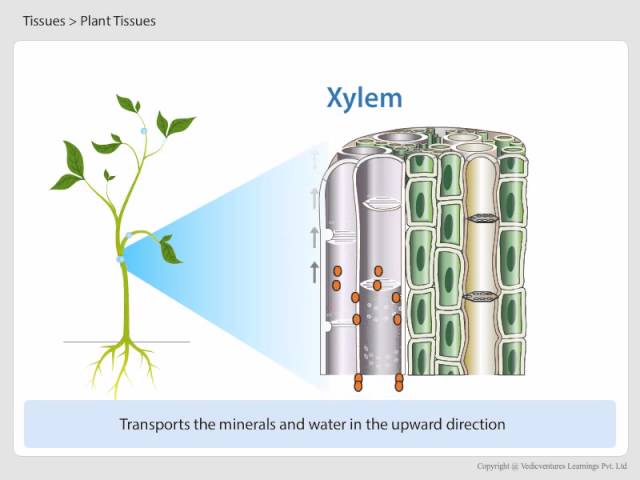The image is a detailed diagram of a plant taken from a manual or book, set against a white background with a light gray border. On the top left corner, in black writing, it reads "Tissues > Plant Tissues." The left side of the diagram features an illustration of a plant stem with leaves and visible roots. A blue light connects the plant to a zoomed-in section on the right, showcasing the internal structures of the stem. This closer view reveals several columns: two transparent ones, seemingly filled with water and adorned with orange dots, and other columns in green and yellow hues, with lines and dark green circles. Above one column, in blue writing, is the label "Xylem," denoting the tissue that transports minerals and water upward. These transport channels are detailed further with little red elements on gray parts and an inscription across the bottom that states "Transports the Minerals and Water in the Upward Direction." The image is completed with a blue rectangular background at the bottom and a small, somewhat blurry note on the lower right corner that reads "Copyright of something-something Learnings, LTD."